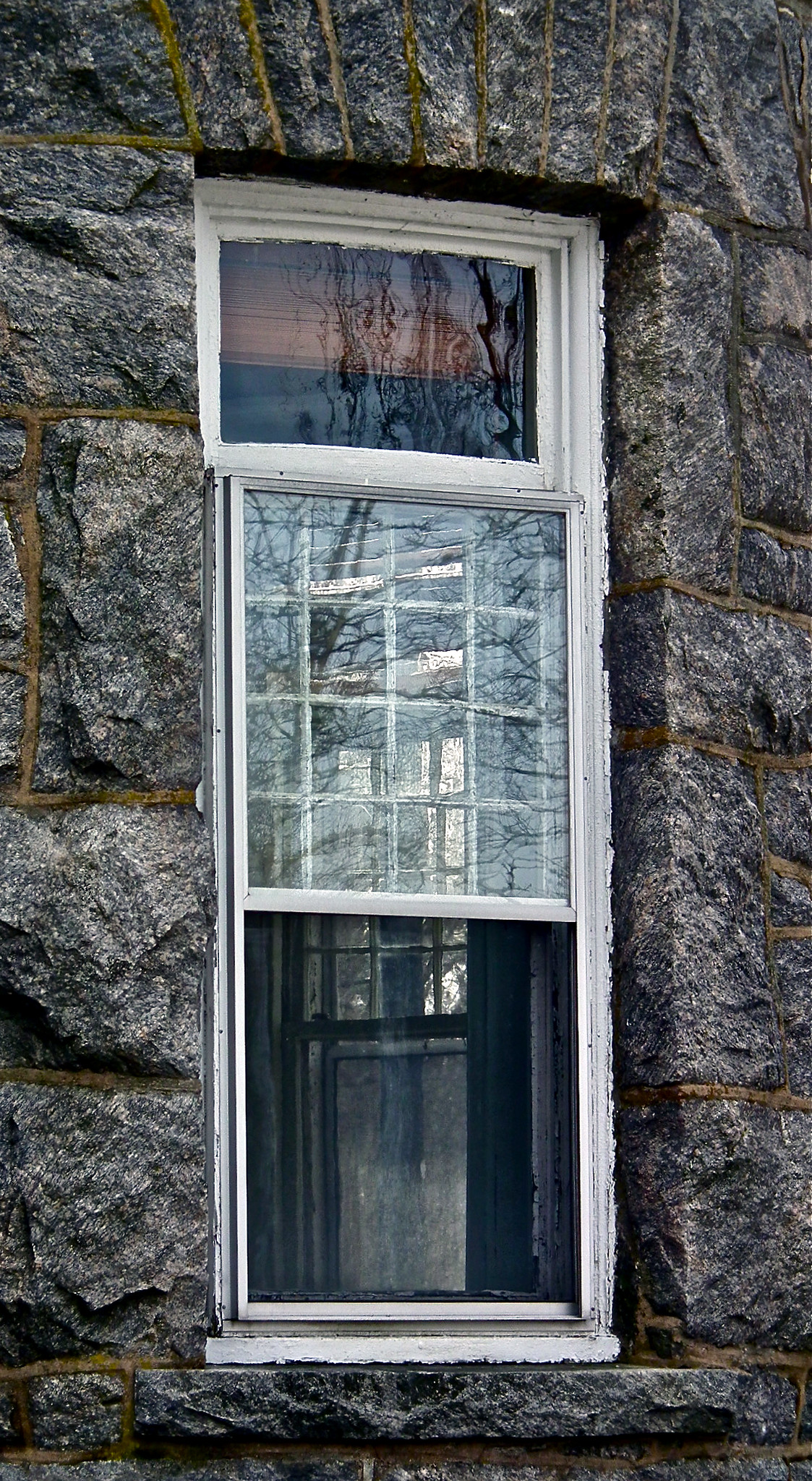This photograph depicts an exterior view of a house constructed with large, dark gray stone bricks, bonded together by yellowish-brown cement. At the center of the image is a tall, modern window framed with white molding. The window is divided into three sections: the top section features a plain glass pane with a reflective surface, showing a smeared reflection of the sky. The middle section consists of a four-by-four grid of smaller square panes, potentially reflecting an adjacent building, while the bottom section is open, providing a glimpse into the dark interior of the house. Inside, you can see another closed window through which a tree trunk, leaves, and some sky are visible. The detailed craftsmanship of the stones gives the structure a castle-like appearance, blending historical architecture with modern window design.